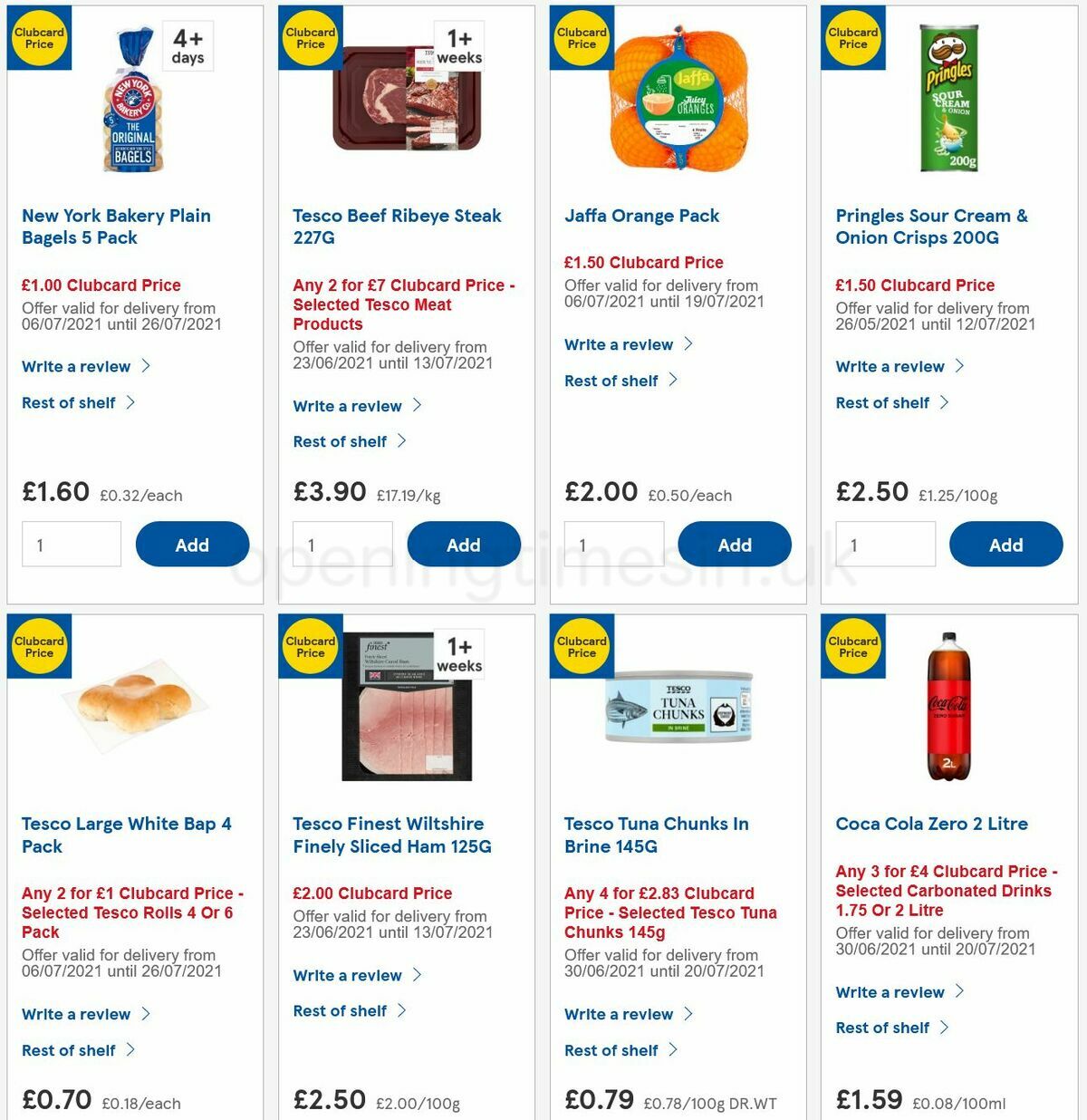The screenshot from the website displays promotional offers for various grocery items against a light gray background. Organized neatly, the image contains two rows, each with four distinct panels.

In the first row:
1. **New York Bakery Plain Bagels Five Pack**: The panel showcases a blue square and a yellow circle adjacent to it, each marked with "Club Card Price," set against a white background.
2. **Tesco Beef Ribeye Steak, 227 G**: The same design elements follow, with the steak item prominently described.
3. **Jaffa Orange Pack**: Highlighting a pack of oranges with the standard layout.
4. **Pringles Sour Cream and Onion Crisps, 200 G**: Featuring the popular snack in familiar packaging.

In the second row:
1. **Tesco Finest Wiltshire Finely Sliced Ham, 125 G**: The panel continues with the finely sliced ham as advertised.
2. **Tesco Tuna Chunks in Brine, 145 G**: Displaying the canned tuna with product-specific details.
3. **Coca-Cola Zero, 2 Liter**: Prominently displaying the soft drink.

Each panel includes an option to "write a review" as well as a link labeled "rest of the shelf." Furthermore, the price of each item is provided in British pounds, and each product is visually represented with its respective image to ensure clarity and easy identification for the consumer.